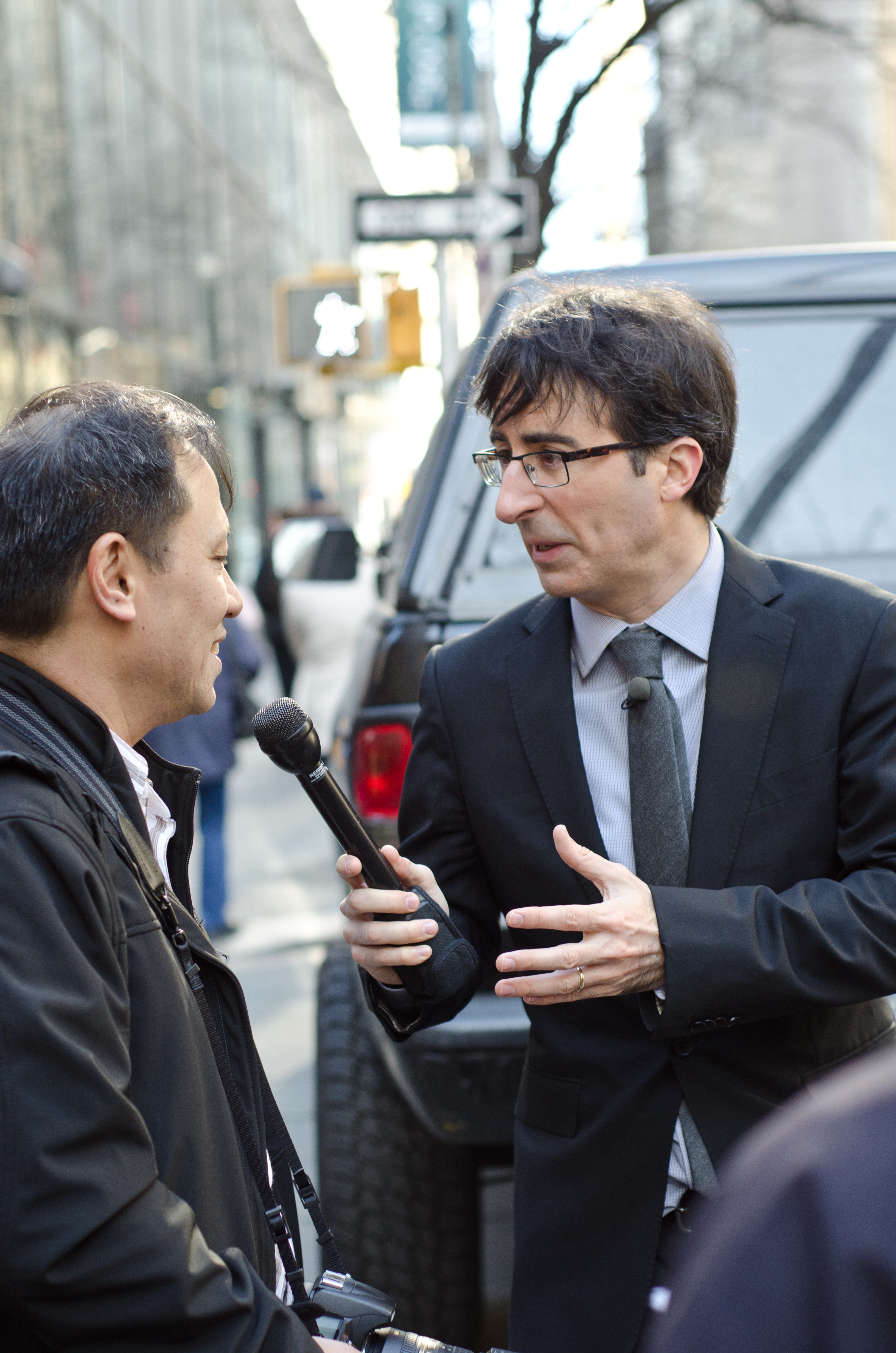In this photograph, we observe two men engaged in a conversation on what appears to be a street side with an urban background. The man on the right, who fits the description of John Oliver, famous from "The Daily Show" and his HBO series, is a white male with dark, shaggy hair and dark-framed glasses. He is dressed in a dark suit jacket, a light blue to gray button-down shirt, and a gray tie. John Oliver is holding a black microphone up to the man on the left. 

The man on the left, an older male of Asian descent with short, dark hair, is wearing a black jacket with a strap bearing a large camera around his neck. He appears to be in mid-sentence, smiling and speaking into the microphone held by John Oliver.

Behind them, there is a dark-colored vehicle, possibly a black SUV or a jeep, and street signs including a blurry black and white one-way sign and a no-walking sign. Further in the background, we can discern blurry tall buildings, suggesting an urban environment. The overall scene suggests an interview or casual conversation taking place outdoors, with John Oliver capturing the moment.